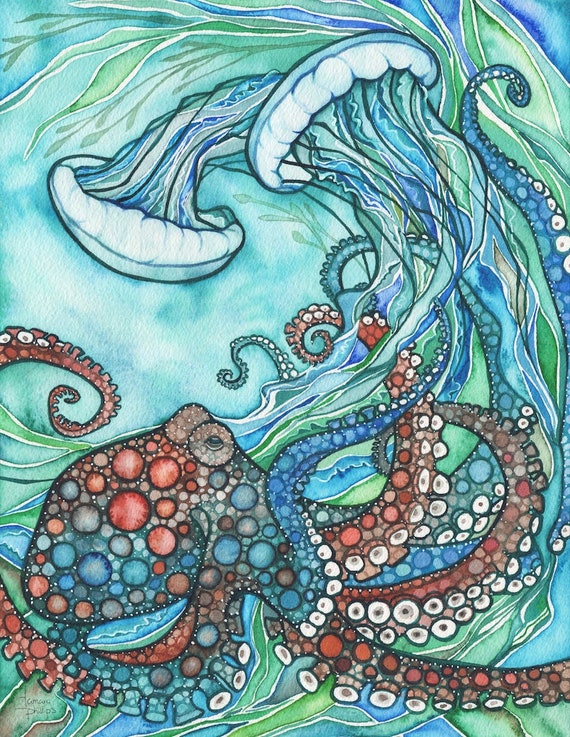This art piece is a vibrant and psychedelic illustration depicting an abstract underwater scene. Dominating the bottom of the vertical image is a fantastical octopus, adorned with swirling tentacles covered in white suction cups. The octopus is rendered in a kaleidoscope of browns, reds, blues, and purples with circular patterns decorating its body, giving it a surreal appearance. Surrounding the octopus are numerous circular motifs and white dots, enhancing the otherworldly quality of the scene.

Floating above are several sea creatures with mushroom-like caps that could be interpreted as jellyfish. These creatures and the octopus are outlined in black, with the interiors filled with softer, faded hues suggestive of watercolor techniques—a blend of gentle blues, greens, and purples. The background is a harmonious mix of blue, green, and whitish tones, perhaps representing an abstract seascape, with streaky green elements resembling seaweed or underwater plants. The overall effect is an imaginative and artistic representation of a marine environment, blending realism with fanciful artistry.